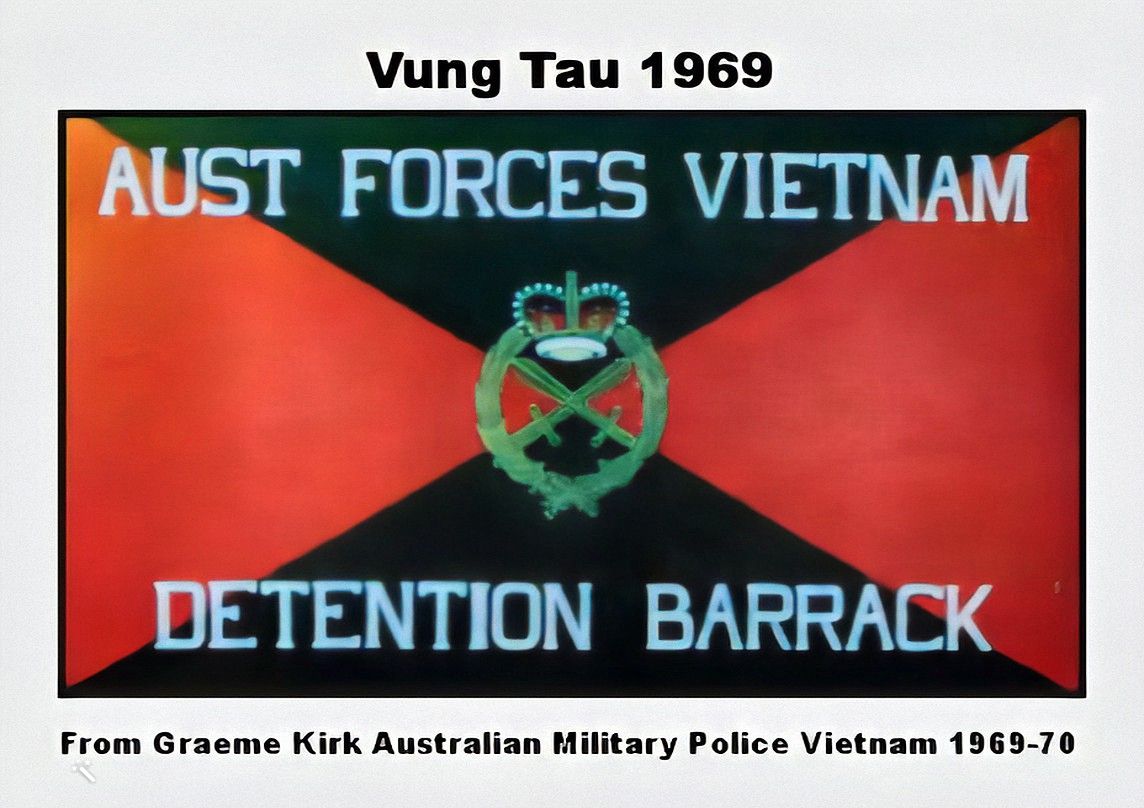The image features a rectangular flag with a silver-gray border, wider than it is tall. The flag is split into four two-colored triangles by an X, with black triangles at the top and bottom, and red triangles on the left and right. In the center of the flag, where the triangles meet, there is an insignia consisting of a green wreath with two crossed swords and a crown atop. At the top and bottom of the flag, in bold gray letters, it reads "Aust Forces Vietnam" and "Detention Barrack," respectively. Above and below the flag, the text on the gray background states, "Vung Tau 1969," and "From Graeme Kirk, Australian Military Police, Vietnam 1969-70." This suggests that the flag might have been used at the Australian Forces Vietnam Detention Barrack in Vung Tau during the mentioned years.